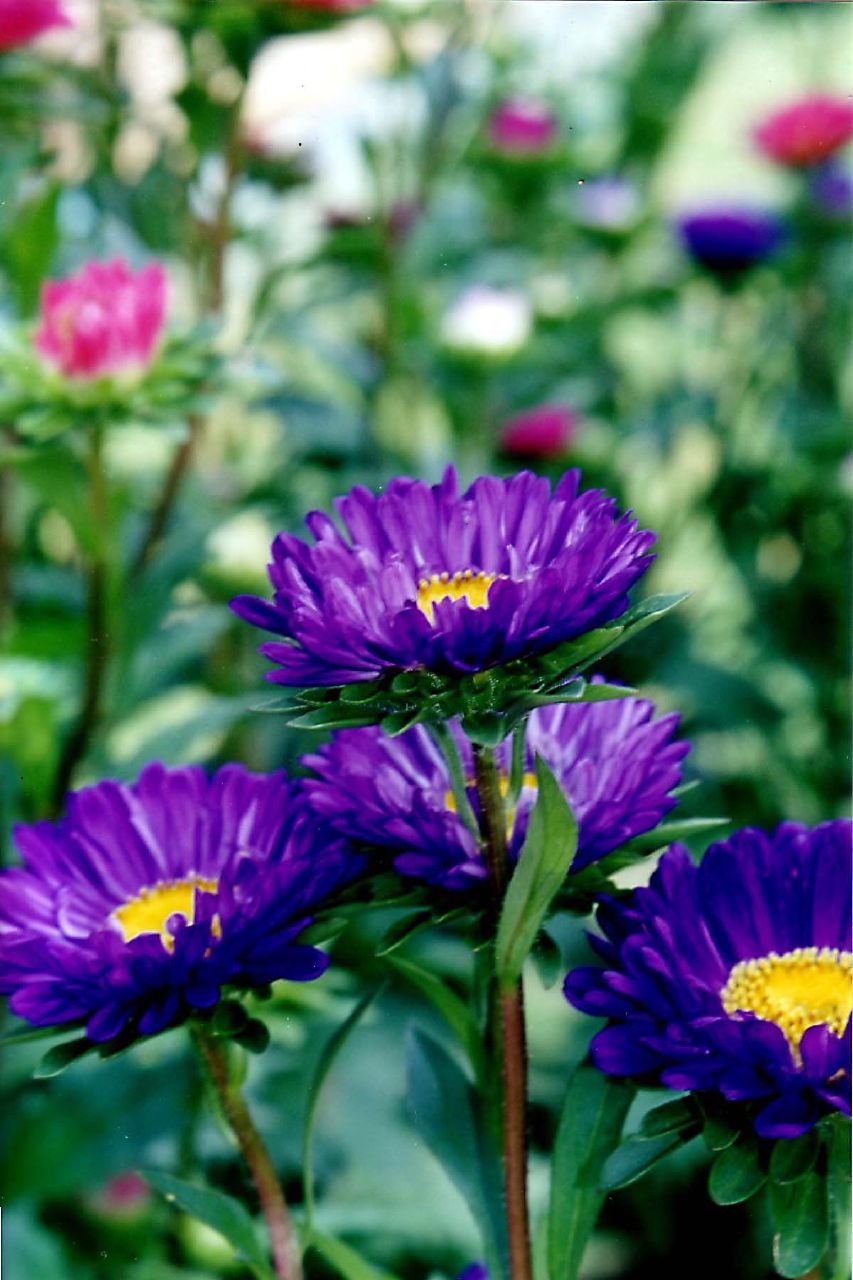This photograph features a vibrant floral scene most likely captured in the middle of a prairie or garden. The image centers on four prominent purple flowers with striking marigold-yellow interiors and brown stems, each detailed with individual petals. These flowers stand out clearly against the blurred background, which is rich in greenery. Scattered throughout the background are at least six additional flowers in varying shades of pink and purple, providing a colorful tapestry. A notably taller purple flower stands to the rear with similar characteristics to those in the foreground. Sunlight filters through this lush setting, adding a natural glow to the scene. Laden with green stems and leaves, the background hints at an abundant, thriving outdoor environment.